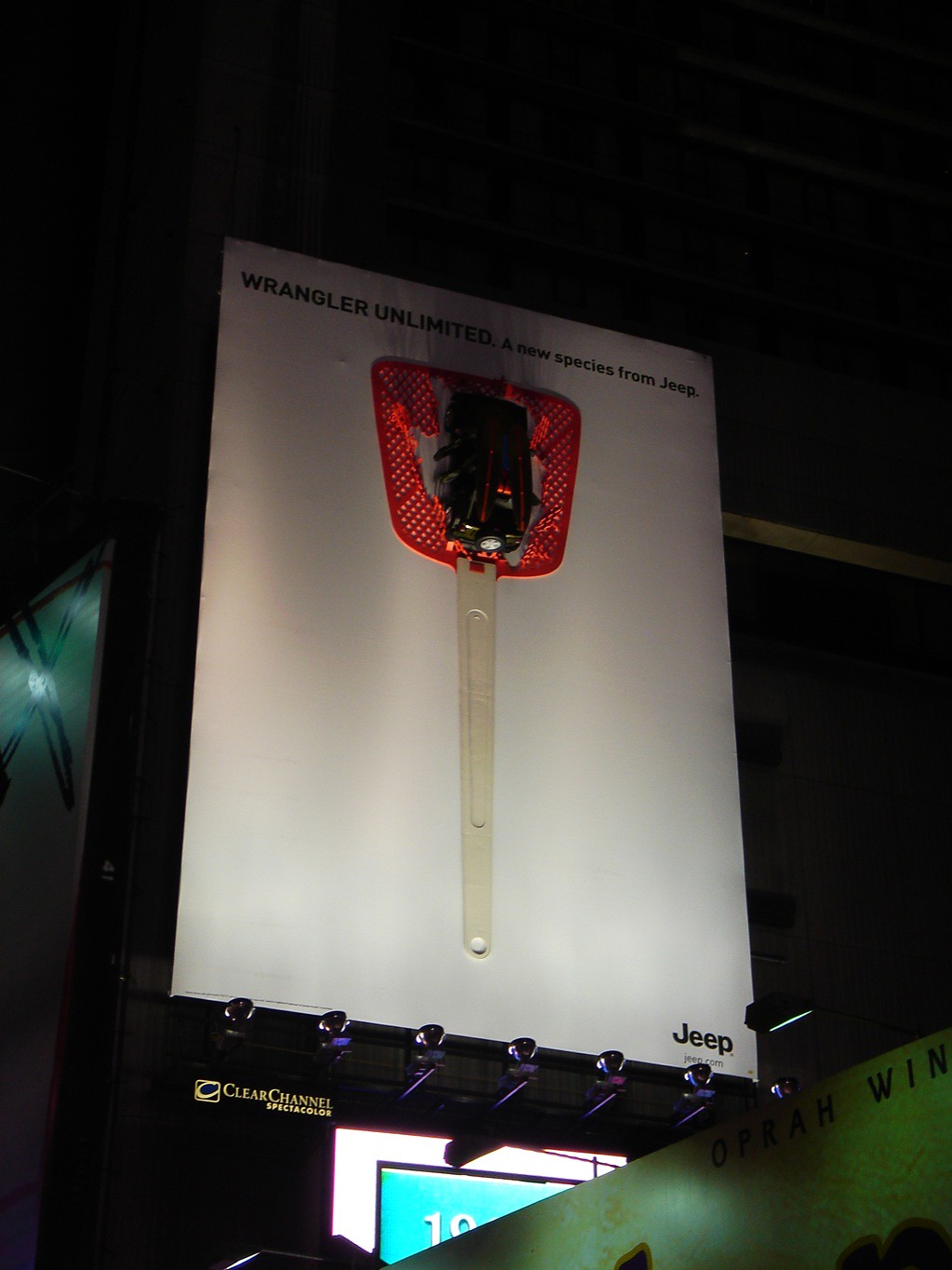In this high-quality nighttime photo, the main focus is a large, prominently displayed Jeep billboard against a dark sky. The top of the billboard reads, "Wrangler Unlimited, a new species from Jeep." A striking three-dimensional display features a beige-handled, red-webbed fly swatter broken in the middle, with a black Jeep Wrangler model seemingly bursting through it, creating the illusion that the vehicle has smashed through the swatter. At the bottom right of the billboard, the Jeep logo is clearly visible. The lighting emphasizes the billboard despite the night setting. The surrounding scene includes some nearby buildings and other billboards, but the Jeep advertisement remains the central highlight.